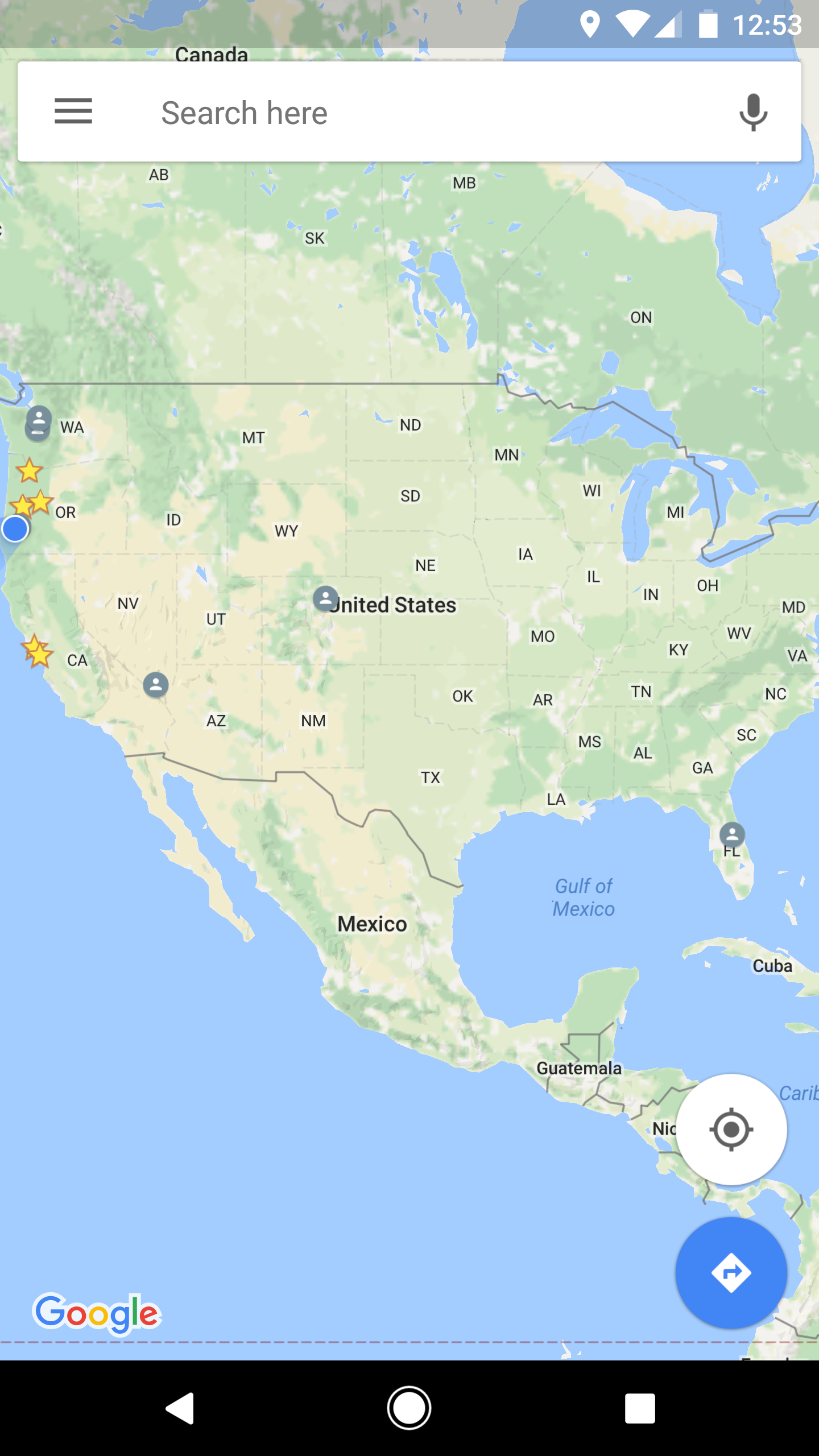A highly detailed map of the United States is displayed, with the land areas portrayed in shades of green and gray. Above the U.S., the neighboring country of Canada is visible, while Mexico, Guatemala, and Nicaragua are depicted to the south. The map features a top search bar labeled "search here." In California, there are four locations marked with yellow stars. There is a special point of interest highlighted by a blue circle on the map. Geographical features such as the Great Lakes and the Gulf of Mexico are clearly depicted, along with portions of the Pacific Ocean. Each state is identified by its two-letter abbreviation. Across the middle of the map, the text "United States" is prominently displayed. In the lower right corner, there are two circles: a white one, likely for zooming in on specific regions, and a blue one with an unspecified function.